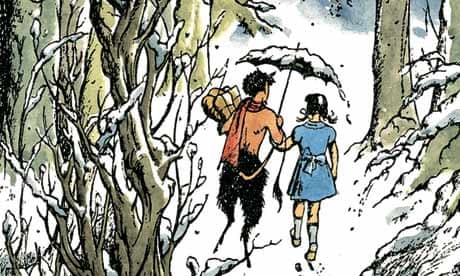In this detailed, vibrant illustration, a snowy forest unfolds, showcasing a touching scene evocative of a children's storybook, possibly from "The Lion, the Witch, and the Wardrobe." Centered in the composition, a satyr and a young girl walk forward with their backs towards us, creating a poignant and whimsical moment. The satyr, characterized by his goat-like legs, hooves, and black horns, sports dark fur and a flowing reddish scarf, and he carries a collection of packages in his left hand. Holding a snow-dusted black umbrella in his right hand, he tenderly escorts the little girl, who intertwines her arm with his. She’s dressed in a blue outfit adorned with a ribbon on the back, white high socks, and shoes, her dark hair styled in braids. The snowy path they tread is framed by snow-laden branches on either side, adding a serene winter backdrop to this enchanting scene. The satyr’s gentle guiding presence contrasts with the crisp and quiet woodland, making the illustration both heartwarming and magical.